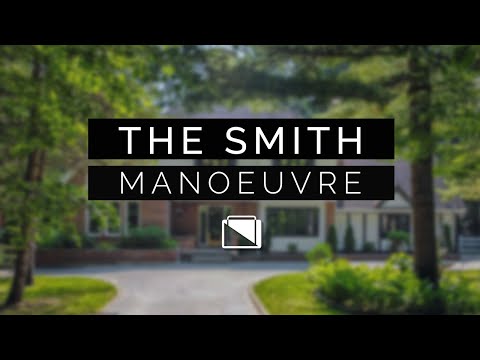The thumbnail image for "The Smith Maneuver" prominently features a suburban house as the blurred background. This house combines red brick on the left side and white siding on the right, and it's topped with a black roof. A well-maintained driveway runs up the center, flanked by vibrant green trees on both sides, and further surrounded by neat hedges and bushes. The foreground is dominated by two horizontal black bars—one at the top and another at the bottom—framing the image with a wide-screen appearance. Within these bars, white text bears the words "The Smith Maneuver." Additionally, a transparent white icon resembling a suitcase or briefcase is positioned below the text. The entire composition gives a sense of a polished, professional presentation, possibly for a video or a slide.